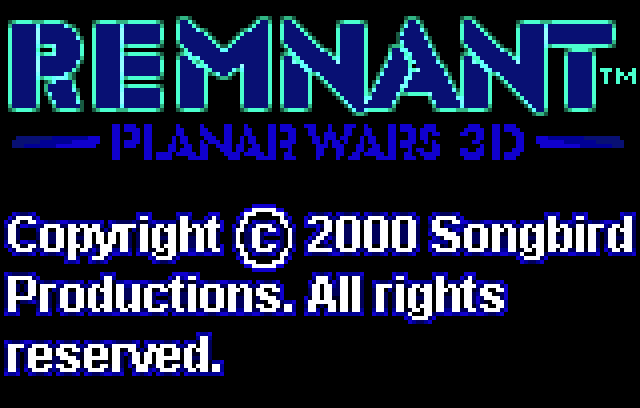The image features a black background with a digitized and pixelated text that resembles the cover art of a video game. At the top, in large, bright blue letters outlined in a neon teal color, the title "Remnant™" appears prominently. Below this, in slightly smaller bright blue letters, "Planar Wars 3D" is displayed, with a sizeable hyphen before "Planar" and after "3D." Further down, in white letters outlined in blue, it reads "Copyright © 2000 Songbird Productions. All rights reserved." The overall style conveys a futuristic, sci-fi theme.